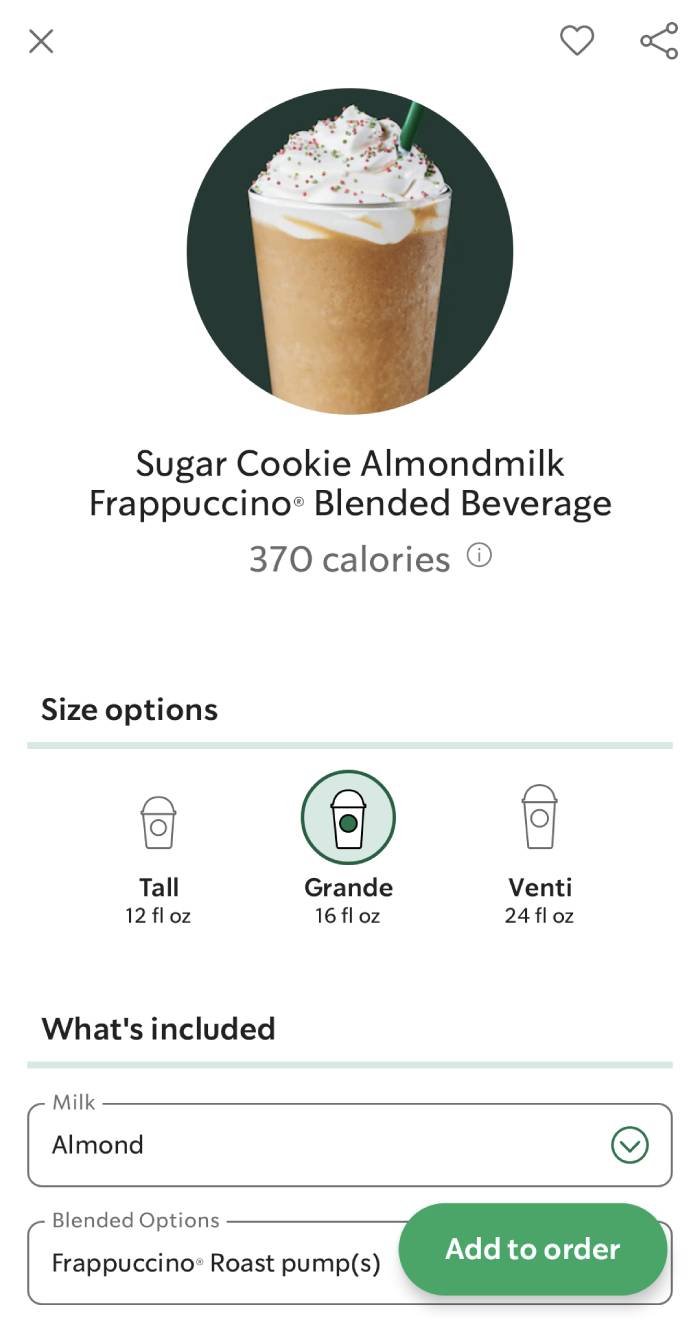A screenshot of the Starbucks mobile app interface displaying a customized beverage order. The background is predominantly green, with a large central icon depicting a latte or blended coffee drink topped with whipped cream, rainbow sprinkles, and a green straw. The top of the screen features navigational options including a close ("X") button on the left, and heart and share icons on the upper right.

Beneath the central icon, text reads: "Sugar Cookie Almond Milk Frappuccino Blended Beverage," along with nutritional information stating "370 calories." The app offers size options for the drink: Tall (12 fl oz), Grande (16 fl oz), and Venti (24 fl oz). The Grande size is currently selected, highlighted by a green circle.

Further customization details indicate the use of almond milk for the beverage, with an option to change the type of milk. Under "Blended Options," selections are shown for "Frappuccino Roast Pump," marked with "S" and apostrophes, suggesting quantity adjustments. 

A prominent light green "Add to Order" button at the bottom hints at the final step to confirm the addition of this beverage to the user's order. The arrangement and design of the interface suggest user-friendliness and ease of navigation, typical of the Starbucks app experience.